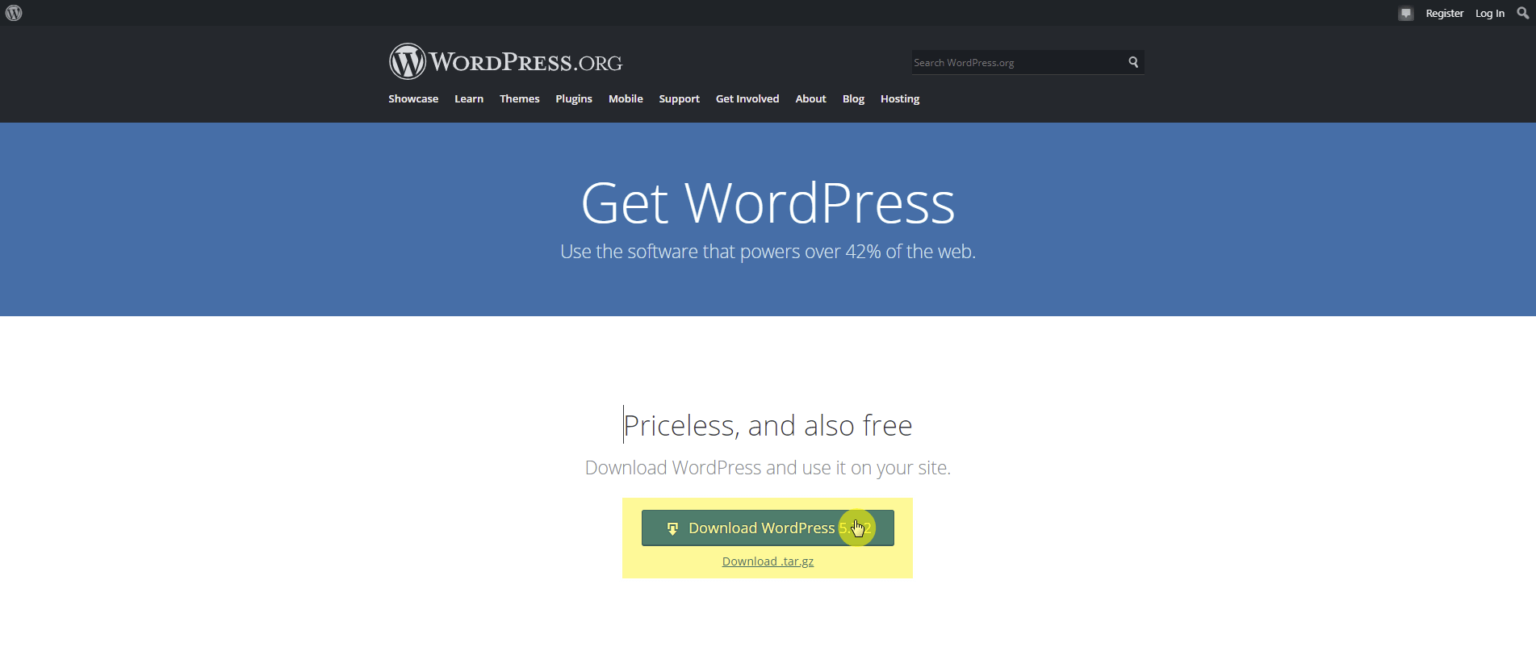The image showcases a section of the WordPress.org website, distinguished by a three-tone color scheme. The top third of the site is black, the middle third is blue, and the bottom third is white. Positioned in the top-center-left area of the black section is the WordPress logo, which consists of a black "W" within a white circle. To the far left of this logo, the words "WordPress.org" are prominently displayed.

In the blue middle section, there's a call to action that reads, "Get WordPress: Use the software that powers over 42% of the web." Below this, in the white bottom section, more text describes the software, stating, "Priceless and also free. Download WordPress and use it on your site." A yellow rectangular button with a green icon is placed below this text, inviting users to "Download WordPress" with a simple click.